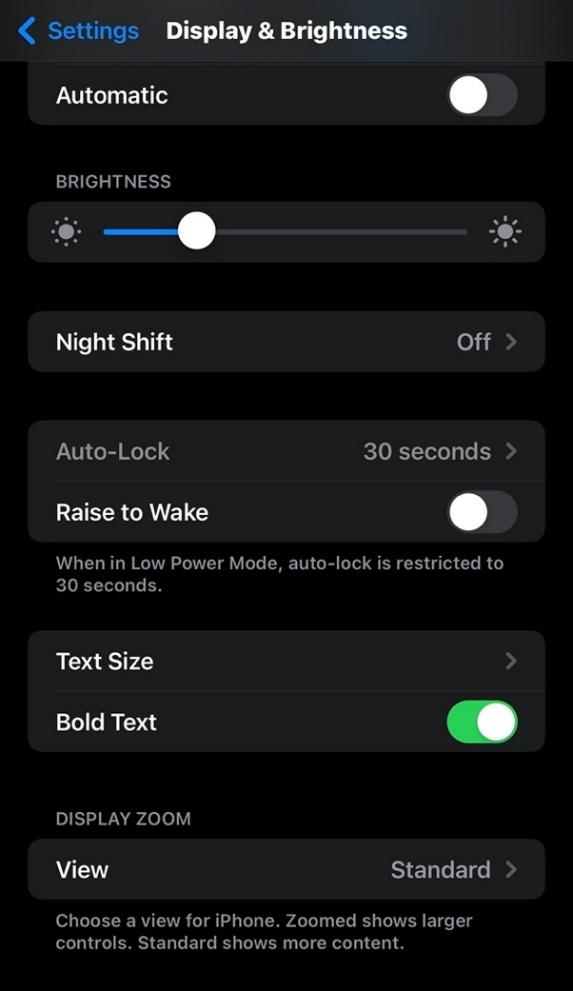Screenshot of an iPhone Settings App: 

At the top of the screen, there's a blue caret for navigating back, with the word "Settings" displayed in blue. Centered at the top of the panel is the heading "Display & Brightness". The background is black, and each setting is presented in dark gray fields.

1. **Automatic**: This option, presumably for automatically adjusting brightness, is turned off.
2. **Brightness**: There's a manual slider set at approximately 30% brightness.
3. **Night Shift**: Designed to filter out blue light, this feature is currently off.
4. **Auto-Lock**: Set to "30 seconds".
5. **Raise to Wake**: Turned off.
6. **Low Power Mode Auto-Lock**: Mentioning that Auto-Lock is restricted to 30 seconds when in Low Power Mode.
7. **Text Size**: Has a caret for further adjustments, but the current size is not specified.
8. **Bold Text**: Turned on.
9. **Display Zoom**: 
   - Currently set to "Standard".
   - Allows users to choose between "Standard" and "Zoomed" views for larger controls or more content on the screen.
   - An explanatory text at the bottom describes: "Choose a view for iPhone. Zoomed shows larger controls. Standard shows more content."

This detailed depiction captures all the settings and features available under "Display & Brightness" in the screenshot.